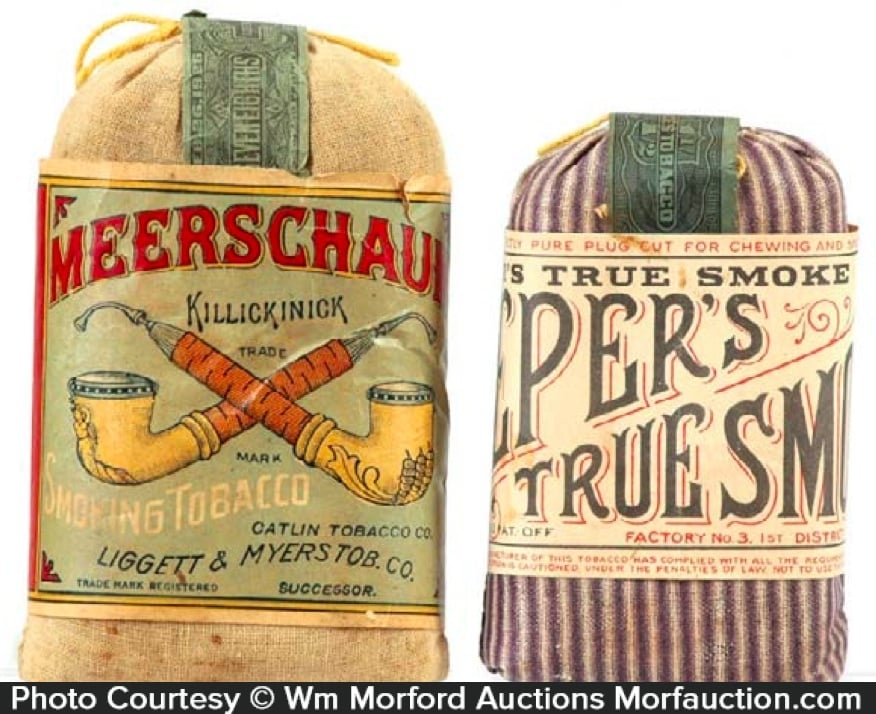The image features a vividly preserved color photograph of two antique tobacco pouches against a white background. At the bottom, there's a black strip with white text that reads, "Photo courtesy of W.M. Morford Auctions, morfordauction.com."

On the left, a cream-colored sack is sealed with a yellow zip tie. The label on this sack reads, "Meerschaum Killing Nick Trademark, Smoking Tobacco, Catlin Tobacco Co., Liggett and Myers Tobco," with a logo featuring two intercrossed pipes. Uniquely, the long end of the pipes resembles carrots with golden-yellow tips where the smoke would emerge.

To the right is a shorter, seersucker-patterned cotton pouch with vertical purple and white stripes. Its label partially reads "Pure Plug Cut for Chewing. True Smoke, Factory Number Three," though some text is obscured. Both labels evoke a vintage, carnival-like presentation.